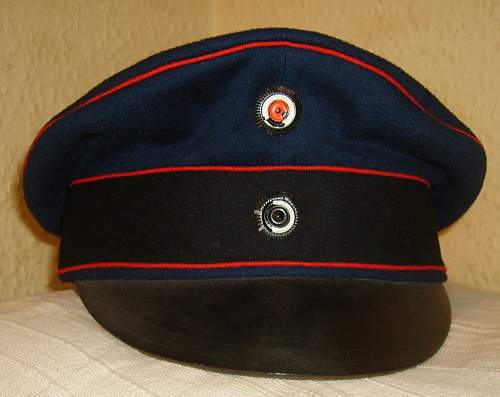The photograph captures a military-style cap positioned on a white, ridged fabric surface that appears to be a bed or a pillow. The background showcases a textured, yellow wall meeting in a corner, adding depth to the setting. The cap itself is primarily dark blue, made of a thick fabric, and features distinctive red piping. It is adorned with a black band around its base, bordered by red piping on both the top and bottom edges. The black bill of the cap is pointed downwards. Noteworthy details include two buttons: one silver button centered on the black band in the front, and another black, white, and red button positioned on the top part of the cap. The overall composition emphasizes the contrast between the dark blue of the hat and the lighter background, highlighting the cap's intricate design elements.